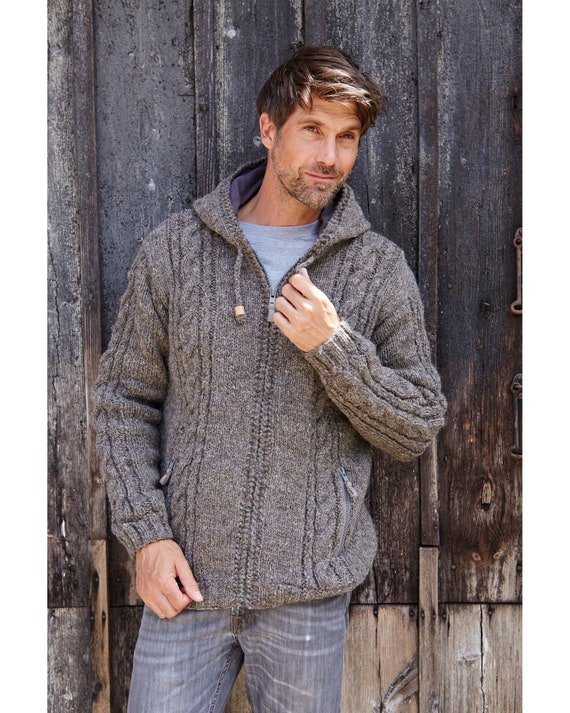This catalog-esque photograph features a white man standing against an aged, weathered wooden wall, its darkened, almost charred appearance highlighting the lighter brown hues at the base. The wood has the look of being quite old, with a texture that tells a story of time and the elements. The man, facing the camera with his head slightly tilted to the right, has short, light to medium brown hair, and a neatly trimmed beard that features hints of gray. His brown eyes glance subtly upwards and to the right. He is dressed in a gray, hooded, cable-knit sweater, with a t-shirt underneath, adding to the layered, textured look. His jeans are light stonewashed blue with distinctive white streaks across the thighs, and have faint creases that add to their worn, yet stylish appearance. One hand rests on his chest area while the other hangs by his side. Bathed partially in the shade of the old fence, a touch of sunlight filters over, subtly illuminating his facial features and upper body.